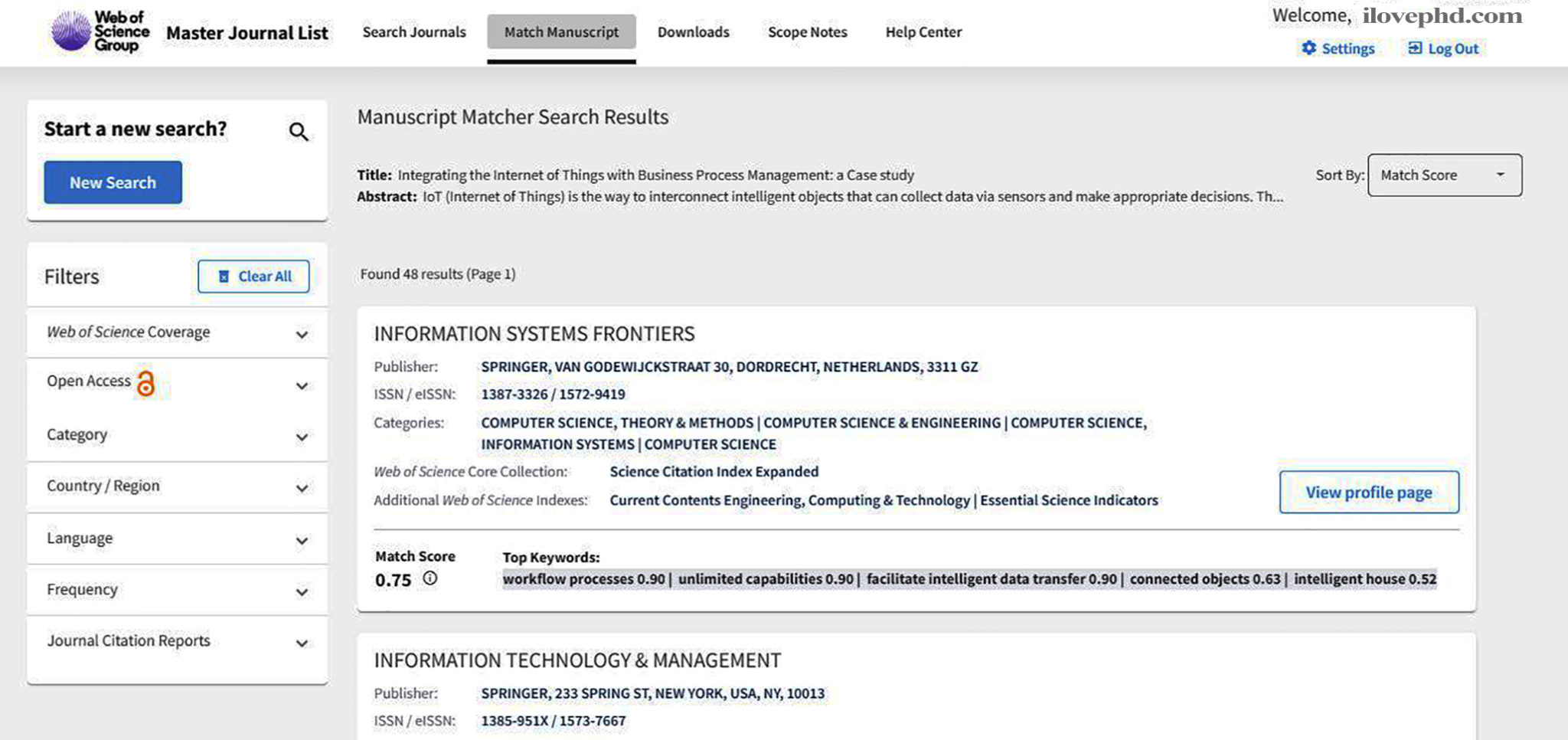The screenshot displays the homepage of the Web of Science group's online platform, being accessed through ilovephd.com. In the upper left-hand corner, a distinctive round purple icon is visible. Immediately to the right, the title "Web of Science Group" is prominently displayed, with "Master Journal List" indicated just below it. A horizontal menu is positioned at the top of the screen, featuring options: "Search Journals," "Match Manuscript," "Downloads," "Scope Notes," and "Help Center."

In the upper right-hand corner, the user is greeted with "welcomeilovephd.com." Below this greeting, a blue widget icon labeled "Settings" is situated, followed by a square icon with a cross that says "Log Out."

To the left side of the screen, a vertical panel allows users to initiate a new search. Various filters are available, including "Web of Science Coverage," "Open Access," "Category," "Country/Region," "Language," "Frequency," and "Journal Citation Reports."

The main portion of the screenshot, centrally located, shows the results of a "Manuscript Matcher" search. One of the highlighted results is titled, "Integrating the Internet of Things with Business Process Management: A Case Study." Its abstract concisely defines IoT (Internet of Things) as a system that interconnects intelligent objects, capable of data collection via sensors and making appropriate decisions based on this data.